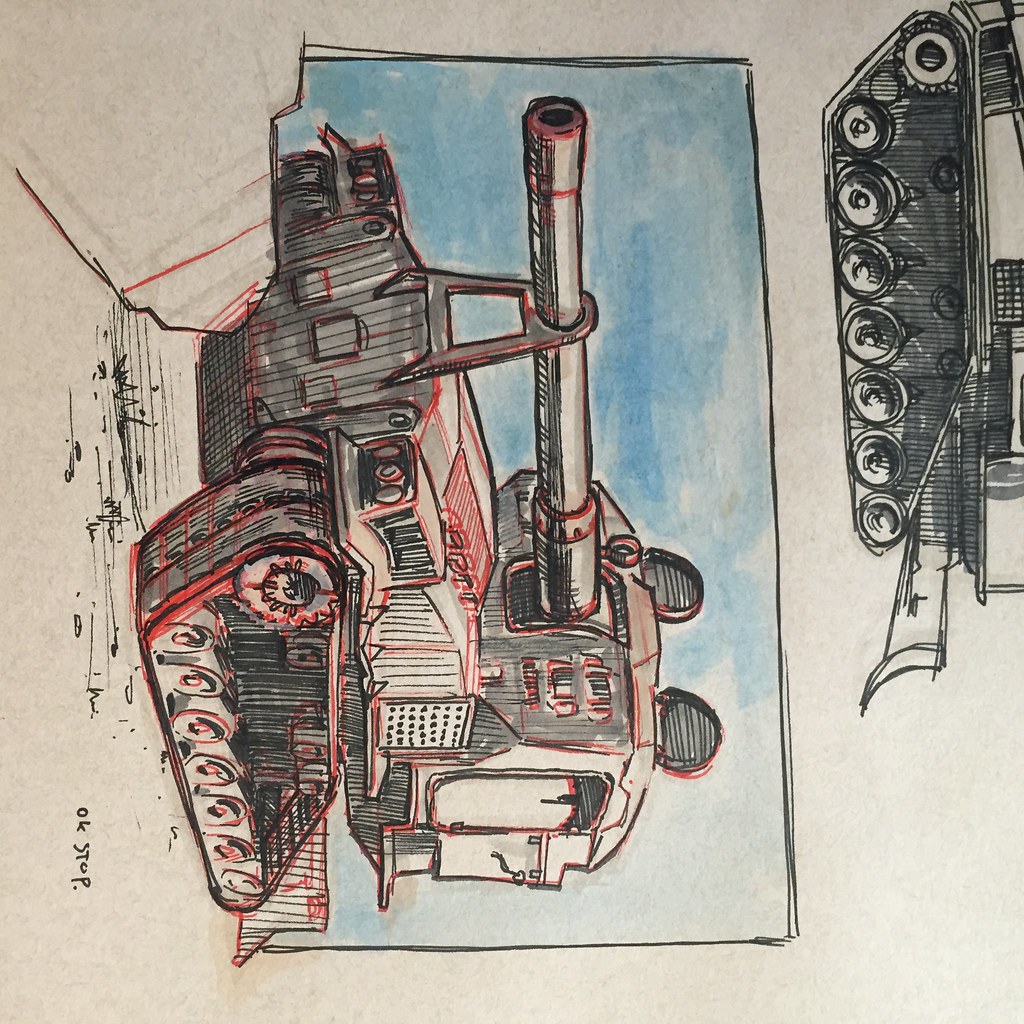This is a highly detailed, high quality portrait-format sketchbook photo featuring a pencil and marker illustration of an old-fashioned, World War II-era tank. The entire image is viewed at a 90-degree angle, causing the tank to appear as if it is pointing upwards instead of to the left. The main image showcases a small tank with a cylindrical barrel extending outwards, poised as if ready to fire. The tank, drawn in sharpie and black marker, is highlighted with red embellishments and set against a light blue, watercolor background. The illustration includes intricate details such as headlights at the top of the tank. Additionally, there is a second, partially cropped image of the same tank, seen from a side cross-section, positioned towards the top left, enhancing the overall depth and perspective of the artwork.